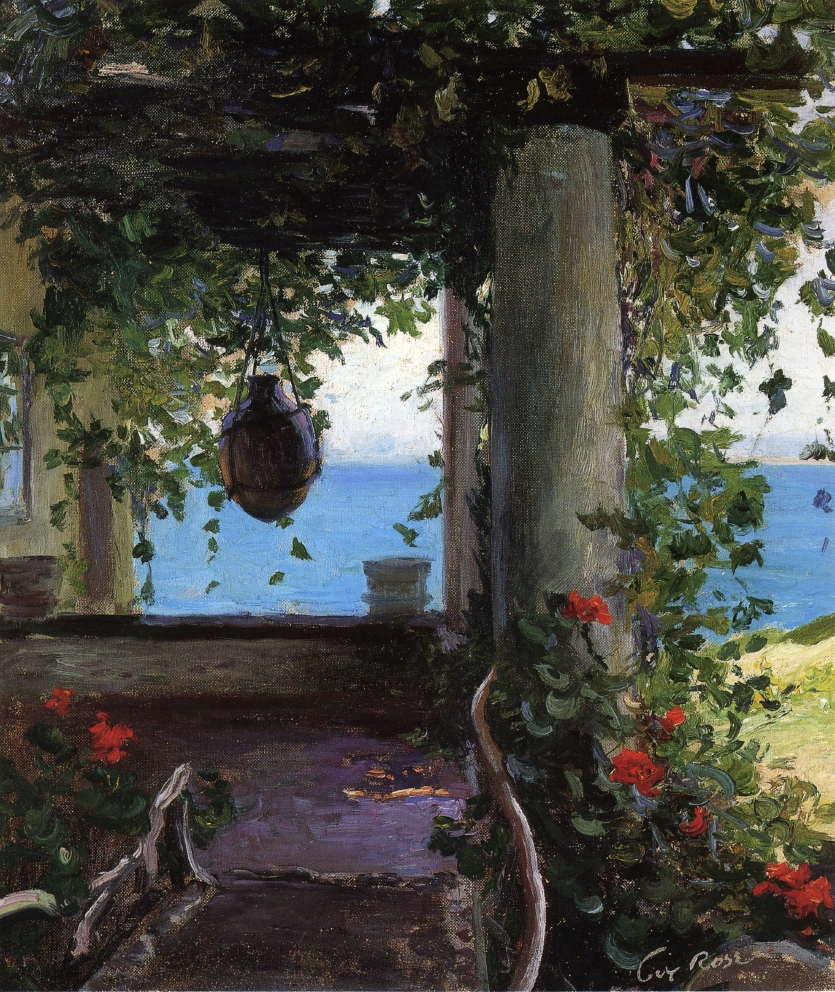This painting by Guy Rose depicts a serene and bucolic garden scene. In the background, a body of blue water stretches out under a white sky, devoid of the sun. The foreground features a shaded sitting area under a canopy flanked by lush greenery and vibrant red flowers. The canopy, possibly part of a covered porch or garden enclosure, is held up by posts, and an intriguing hanging vase adds a charming detail. To the far right, there is a patch of grass, and further to the left, a suggestion of a building or house. The diverse color palette includes hues of tan, red, green, gray, purple, yellow, blue, lime green, and white, contributing to the painting's vibrant and harmonious composition. The artist's signature, "Guy Rose," is clearly visible in the bottom right corner, confirming the artwork's authenticity.